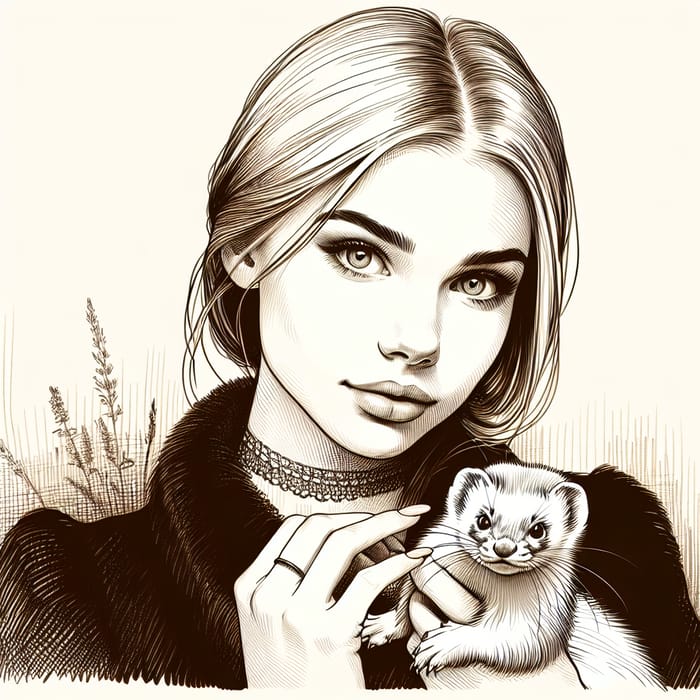This is a highly detailed pen and ink drawing on a cream, off-white background that features a young girl, likely a teenager, with long, center-parted hair that appears blonde in the black-and-white palette. The girl's finely detailed face, with noticeable eye makeup, serves as the focal point of the artwork. She’s adorned in a fur coat, evident by the intricate cross-hatching especially around the shoulders, and wears a lace choker. A ring graces her well-manicured fingers. In one hand, she holds a primarily white ferret with black and gray accents, its finely rendered details capturing an expression of displeasure. The background includes subtle plant growth and flowers, suggesting an outdoor setting, possibly a garden. The fine lines and attention to detail highlight the artist's meticulous style.